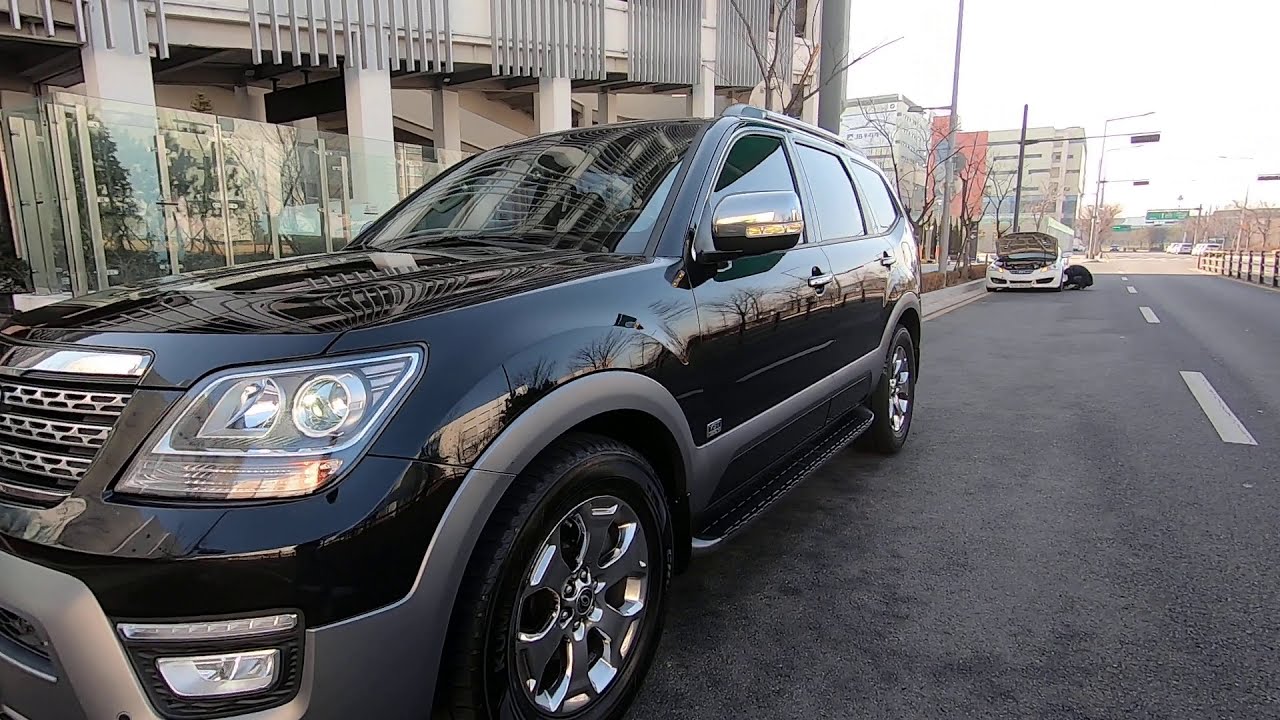A detailed image shows a shiny black SUV with silver hub wheels prominently parked on the side of a dark gray asphalt road, which features a dotted centerline for lane demarcation. The SUV, likely resembling a Trailblazer, is situated in front of a large building that appears to be a parking garage, identifiable by its numerous glass doors at the bottom. Further down the road, there is a white car with its hood open and a person bent over the left front tire, suggesting a possible breakdown. The scene also includes multiple green street signs and traffic lights in the distance, although their exact details are indiscernible. The area is well-lit, indicating a bright and clear daytime setting, and additional buildings, including gray office buildings and a pink structure, are visible further down the road.